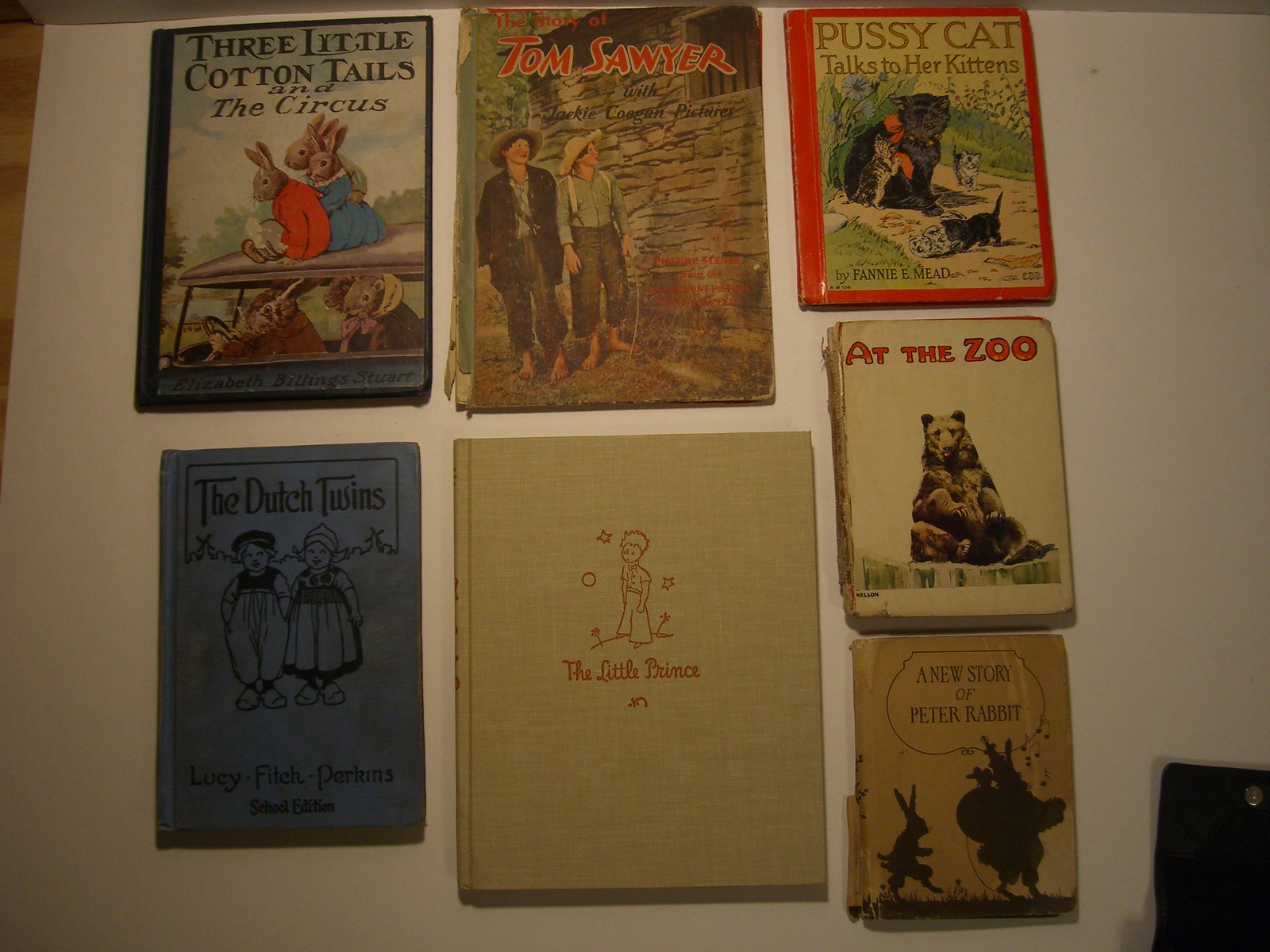This photograph showcases a collection of seven vintage children's books arranged on a light-colored surface, which is overlaying a piece of white poster board. The aged nature of these books is evident through their weathered covers, yellowed pages, and worn bindings. From left to right, the titles include:

1. "Three Little Cotton Tales at the Circus" by Elizabeth Billings Stewart, featuring an illustration of bunnies, one of which is driving a car.
2. "The Story of Tom Sawyer" with Jackie Coogan pictures, displaying two boys in suspenders and hats walking by a building.
3. "Pussycat Talks to Her Kittens" by Fannie E. Mead, showing cats with their kittens.
4. "The Dutch Twins" by Lucy Fitch Perkins, noted as the school edition, depicts a boy and a girl on the cover.
5. "The Little Prince," which has an illustration of a boy standing among stars and flowers.
6. "At the Zoo," presenting an image of a large brown bear or grizzly bear.
7. "A New Story for Peter Rabbit," featuring Peter Rabbit and other elements related to the story.

The vintage condition of these books adds a nostalgic appeal, with details like peeling binders and aged print evident. In the lower right-hand corner of the image, there is an indistinguishable black object that adds an element of mystery to the scene.